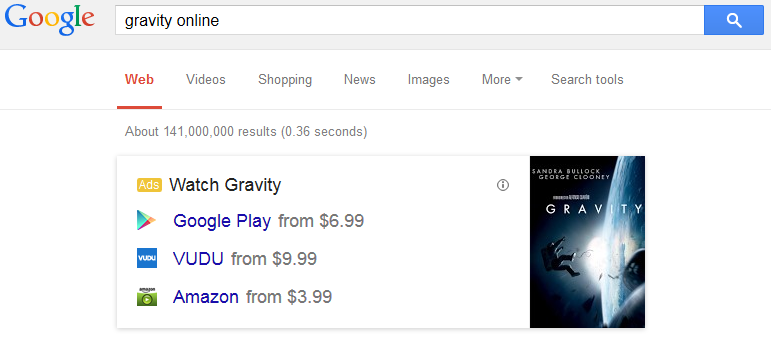A Google search results page is displayed with a primarily white and off-white background. In the upper left corner, the multicolored Google logo is prominently visible. The logo features the letters "G," "o," "o," "g," "l," and "e" in blue, red, yellow, and green. To the right of the logo, the search query "Gravity Online" is typed into the search box. Adjacent to the search box, on the right, is the blue search button featuring a white magnifying glass icon.

Below the search bar, the search results are presented. The word "Web" is highlighted with red text and an underline, indicating the category of the search results. The primary search result pertains to the movie "Gravity." The top result is marked with a yellow "Ads" label, indicating sponsored content. Next to this label, the text "Watch Gravity" is displayed.

Underneath the sponsored result are three links to different platforms where the movie can be watched. The first link is to Google Play, featuring a price tag of $6.99, accompanied by the Google Play logo. The second link directs users to Vudu, with pricing starting at $9.99, and it is accompanied by the Vudu logo. The third link is for Amazon, listing a starting price of $3.99, along with the Amazon logo. Each platform’s logo is positioned to the left of its respective link, ensuring easy identification of the service providers.